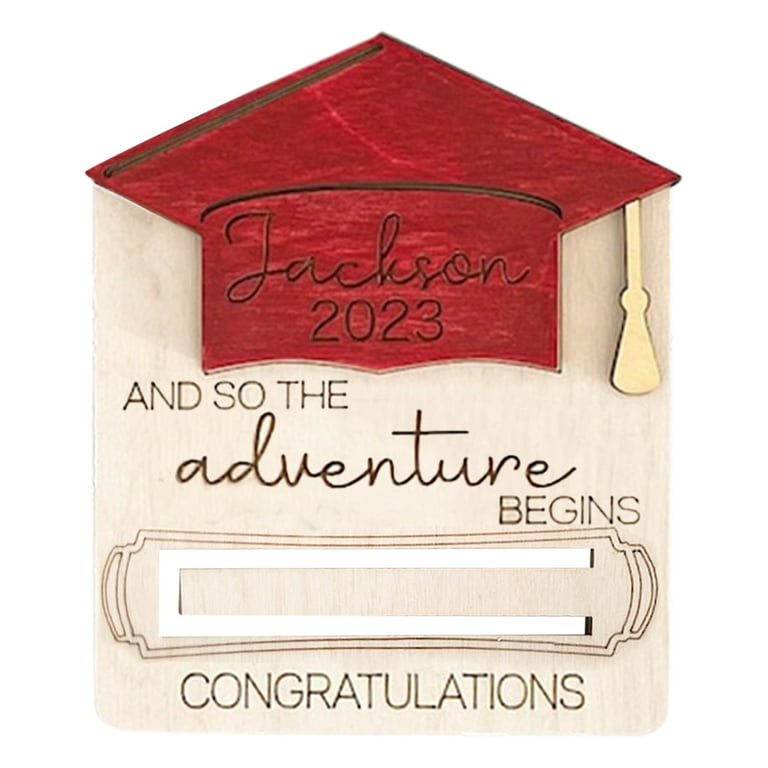The image showcases a meticulously crafted wooden graduation card, primarily light brown with a noticeable grain. Dominating the top is a large red graduation cap, adorned with a golden tassel hanging down. Inscribed on the cap in black font is "Jackson 2023." Below the cap, bold dark brown capital letters declare, "AND SO THE," followed by the word "ADVENTURE" in elegant cursive, and "BEGINS" in smaller capital letters, slightly skewed to the right. A rectangular nameplate-like element is positioned between these phrases and the final line of text. At the very bottom, in bold black capital letters, the card proudly announces, "CONGRATULATIONS." The sturdy wooden material and thoughtful design make this card a unique and cherished memento for Jackson’s 2023 graduation celebration.